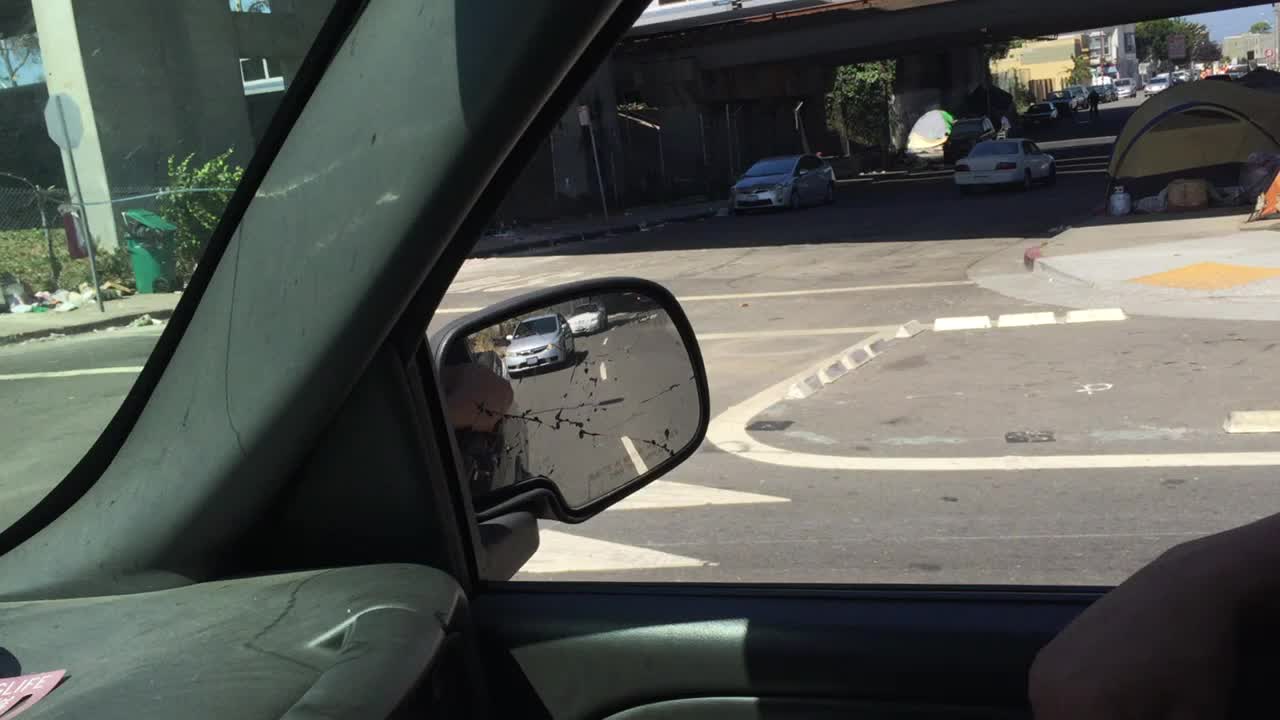This photograph, taken from the front passenger seat of a car, vividly captures an urban scene viewed through the slightly cracked side mirror of the vehicle. The mirror prominently reflects two approaching cars—a silver one directly behind, followed by a white car. The interior of the car is dark gray, with a visible dashboard covered in dust and scattered pieces of paper. Framing the image at the bottom left is the A-pillar, dividing the front and side windows.

Outside the car, the setting reveals a dreary intersection under an overpass, casting a shadow that darkens part of the scene. To the upper right of the image, there is a yellow, rounded tent, suggesting a possible homeless encampment adjacent to the sidewalk. A green, open trash bin is seen near a stop sign, which is directly in the line of sight. The road beneath is gray and marked with white lines, and further off, a grey pillar supports the overpass structure.